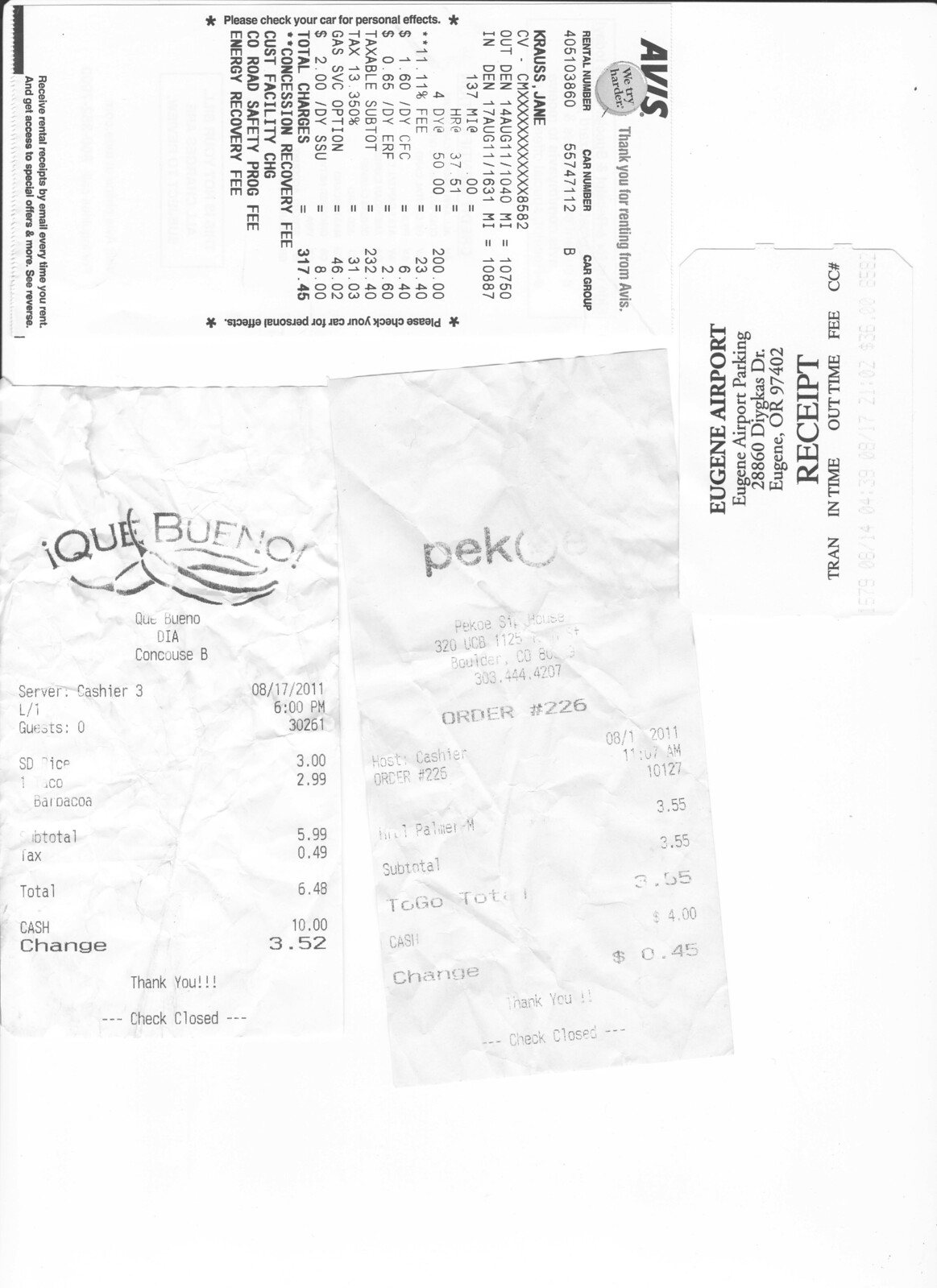The image displays a collection of receipts, likely submitted by a person for work-related expense reimbursement. 

1. **Que Bueno Día at Concourse B (Airport Meal)**:
   - Single receipt in black and white.
   - Details a purchase of a barbacoa taco and a soda.
   - Total amount spent: $3.52.
   - Illustrated with a picture of chilies.

2. **Peko (To-Go Order)**:
   - Receipt is significantly faded, making it difficult to read.
   - Total amount spent: $3.55.

3. **Eugene Airport Parking Receipt**:
   - Only the top part of the receipt is visible.
   - Positioned horizontally.

4. **Avis Rental Cars**:
   - Detailed receipt from Avis Rental Cars.
   - Rental period: August 14th to August 17th (year not specified).
   - Total amount: $317.45.
   - Receipt features the Avis logo and is also positioned horizontally.

The receipts vary in legibility and orientation, with expenses ranging from small food purchases to significant travel-related costs.